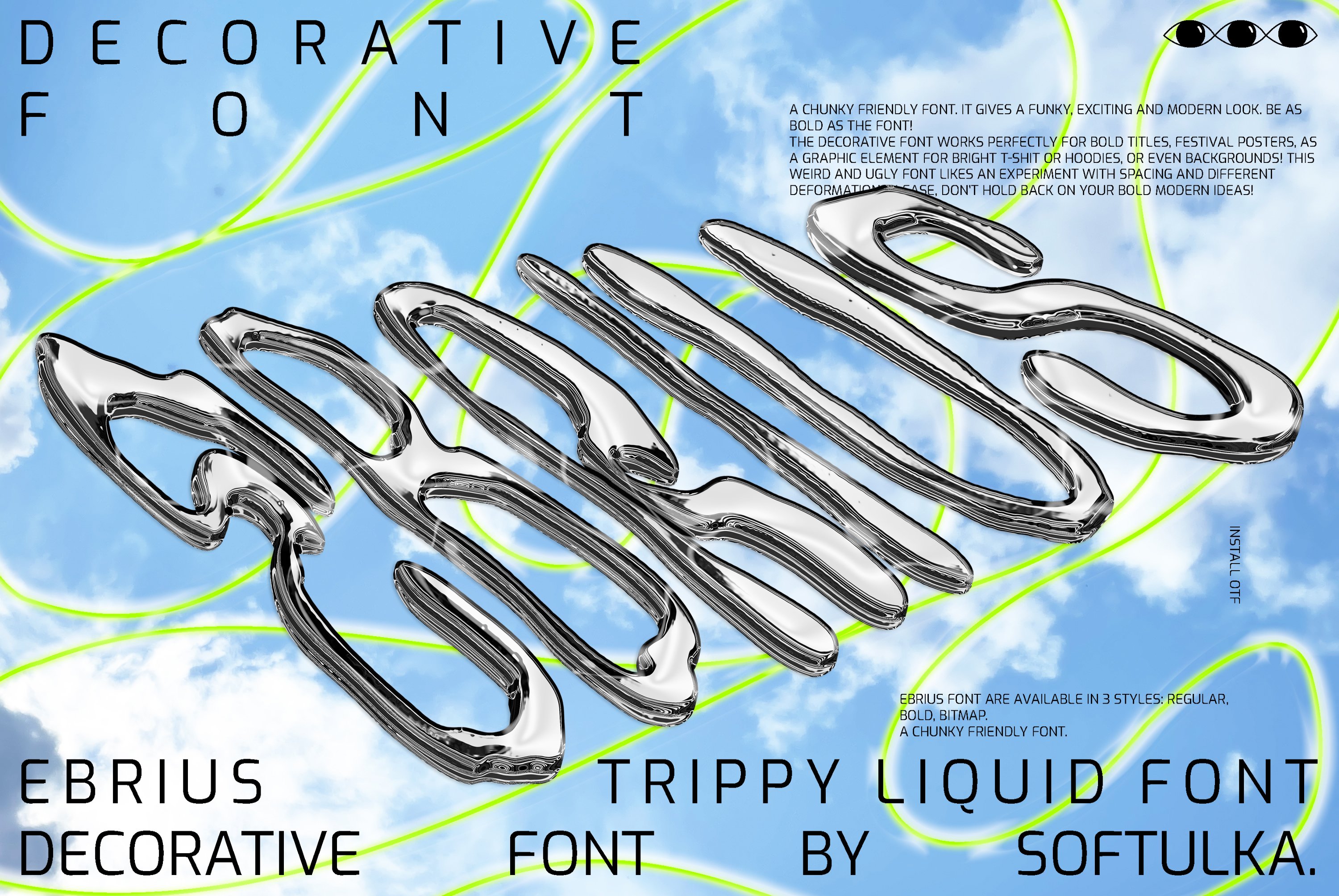This image is an advertisement for the Ebrius decorative font by Softalco. The background features a blue sky adorned with white clouds and a neon green swirl traversing the entire scene, adding a dynamic and trippy effect. In the top left-hand corner, the words "decorative font" are prominently displayed. The Ebrius font itself is showcased in a chunky, liquid, silver style that adds a funky, exciting, and modern look to the image. Described as friendly yet bold, this font is ideal for creating striking titles, festival posters, and graphic elements on bright t-shirts or hoodies, and even experimental backgrounds. The font encourages creativity with its unique spacing and deformative characteristics, urging users to unleash their bold, modern ideas.